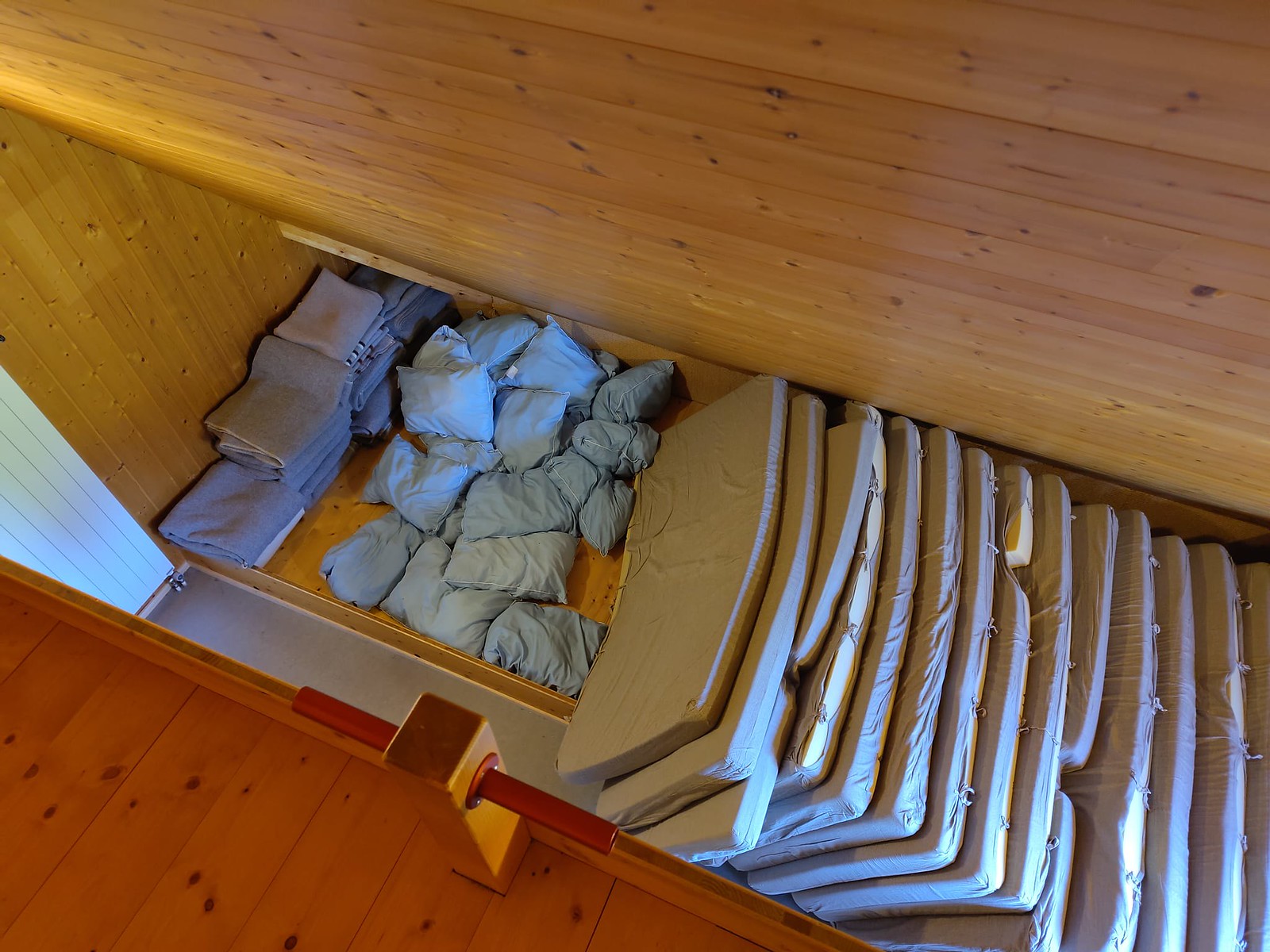The image depicts a wooden-floored area, possibly part of a cabin or campsite. On the right side of the scene, there are numerous gray mattresses or cushions neatly stacked. Nestled beside these are several blue pillows. To the left, blue blankets are folded and piled next to the mattresses and pillows. The room's walls are primarily wooden, with a small section of white wall visible. A wooden banister, adorned with a bit of red paint, separates the viewpoint from the storage area, creating a unique, downward perspective of this cozy, well-organized corner.